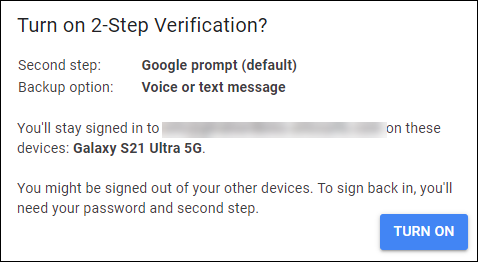The image features a user interface with a clean white background bordered by a thin black line. Dominating the top section, the text "Turn on two-step verification" is prominently displayed in black, large-font type. Directly beneath this, in smaller gray lettering, are the words "Second step," followed by "Google Prompt (default)" in bold black font enclosed in parentheses. 

The next line reads "Backup option" in gray font with "Voice or text message" boldly highlighted beside it in black. Further down, in gray text, the instructions "You'll sign in to [Redacted] on these devices," are succeeded by "Galaxy S21 Ultra 5G" in bold black font. The subsequent section notes in gray, "You might be signed out of your other devices. To sign back in, you'll need your password and second step." 

Finally, the bottom right corner of the screen features a blue button with the text "TURN ON" written in all caps white font.